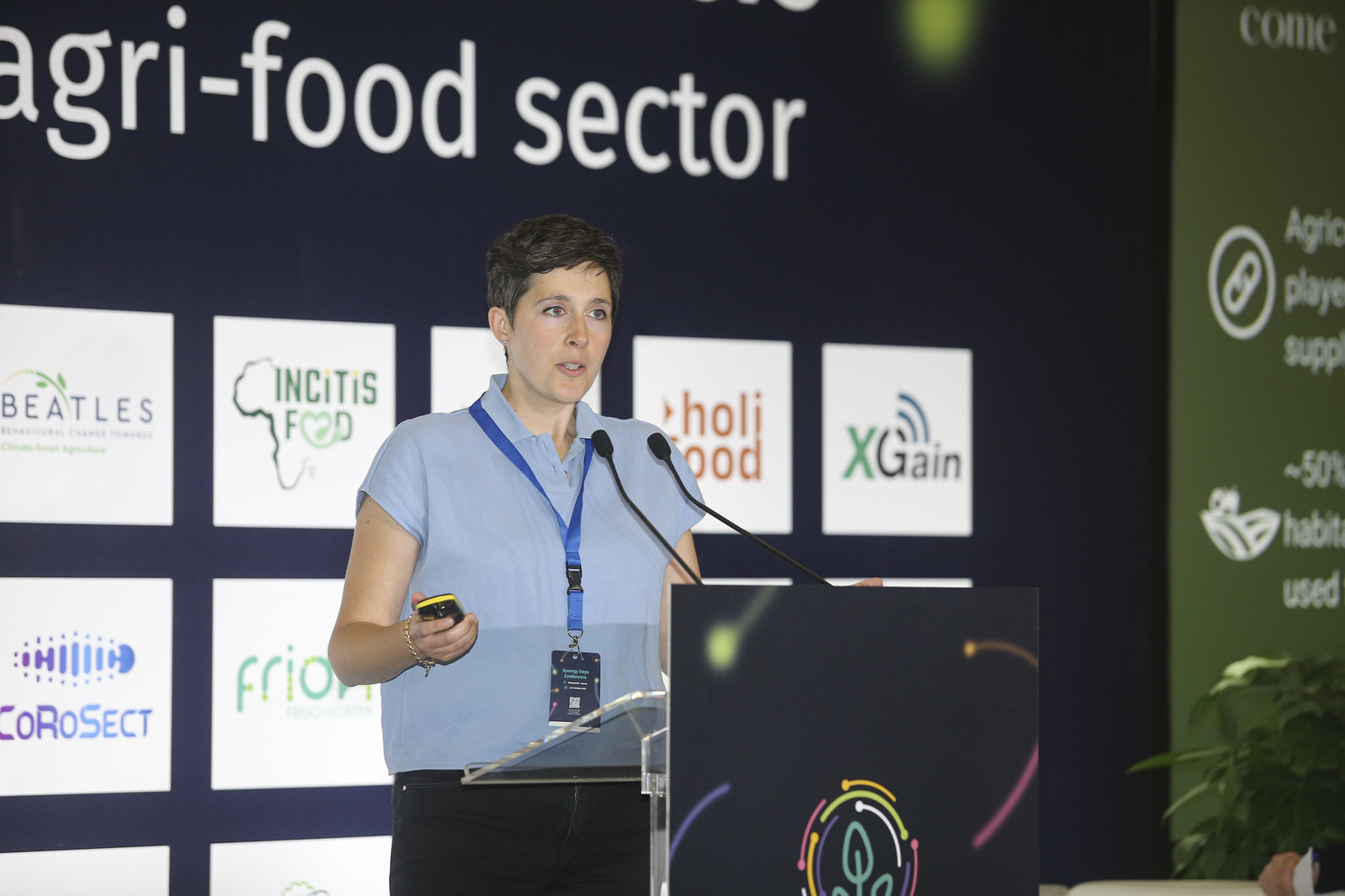In this photorealistic image, a Caucasian woman with short black hair stands confidently behind a glass podium. The podium's front is mostly obscured by a large piece of black paper or cardboard adorned with an intricate array of colorful swirls. At the center of this design is a logo featuring a circular shape filled with hues of pink, green, white, orange, and purple. The woman is dressed in a blue collared t-shirt, black pants, and a blue lanyard that drapes around her neck. In her left hand, she holds a small device with black and yellow coloration. Two black microphones are strategically positioned in front of her, amplifying her voice for the audience. The backdrop behind her is navy blue and includes partially visible white writing, accompanied by a collection of white squares each displaying unique logos or text in various colors like green, orange, and purple. On the right side of the image, a prominent green sign with white text further embellishes the scene.